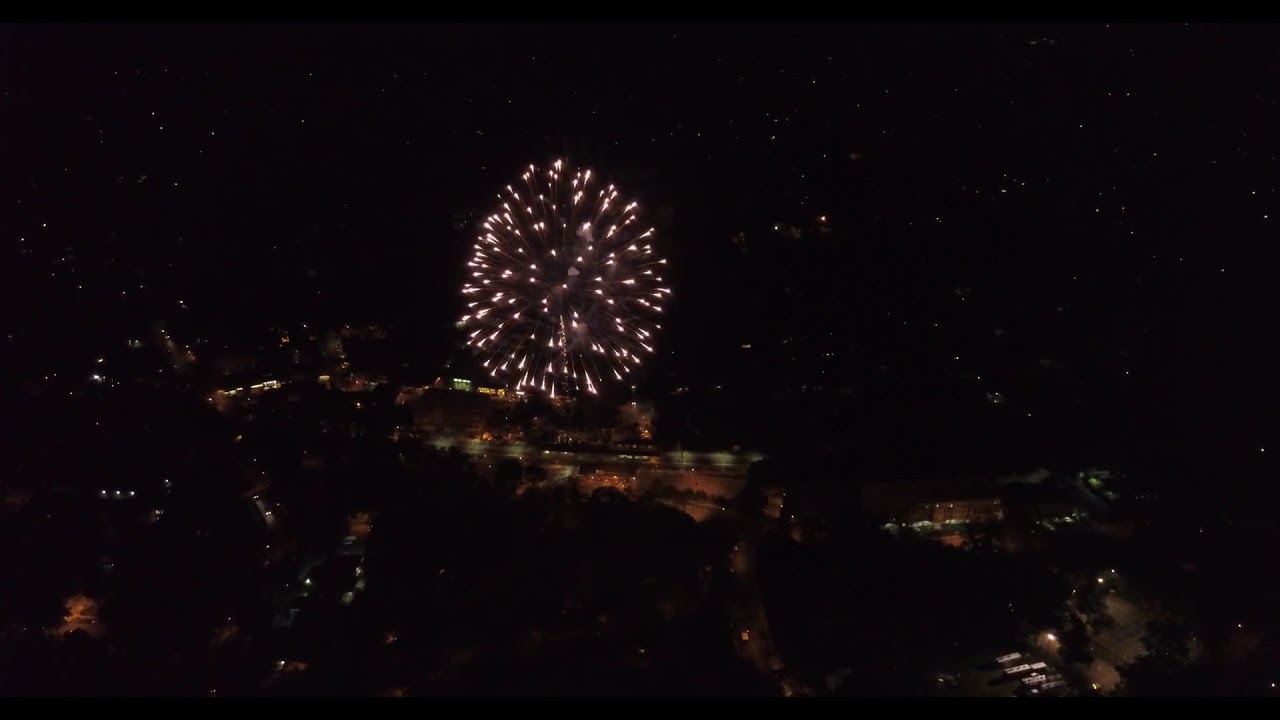This high-definition nighttime photograph captures an impressive overhead view of a firework display. The firework, a large, acorn-shaped burst, shoots out white flames against a deep black sky, lending it a sense of celestial magnificence. Below the central firework, the landscape is illuminated with scattered lights, hinting at a small town or suburb with its low-roofed buildings and street lights. The lights of the structures, possibly commercial, and the faint outlines of vehicles contribute to the image's intricate details. The photograph, slightly blurry, nonetheless captures the essence of a festive night, with the concentrated brilliance of the fireworks in the center framed by the softly twinkling lights of the city below, creating a striking contrast in colors and forms.